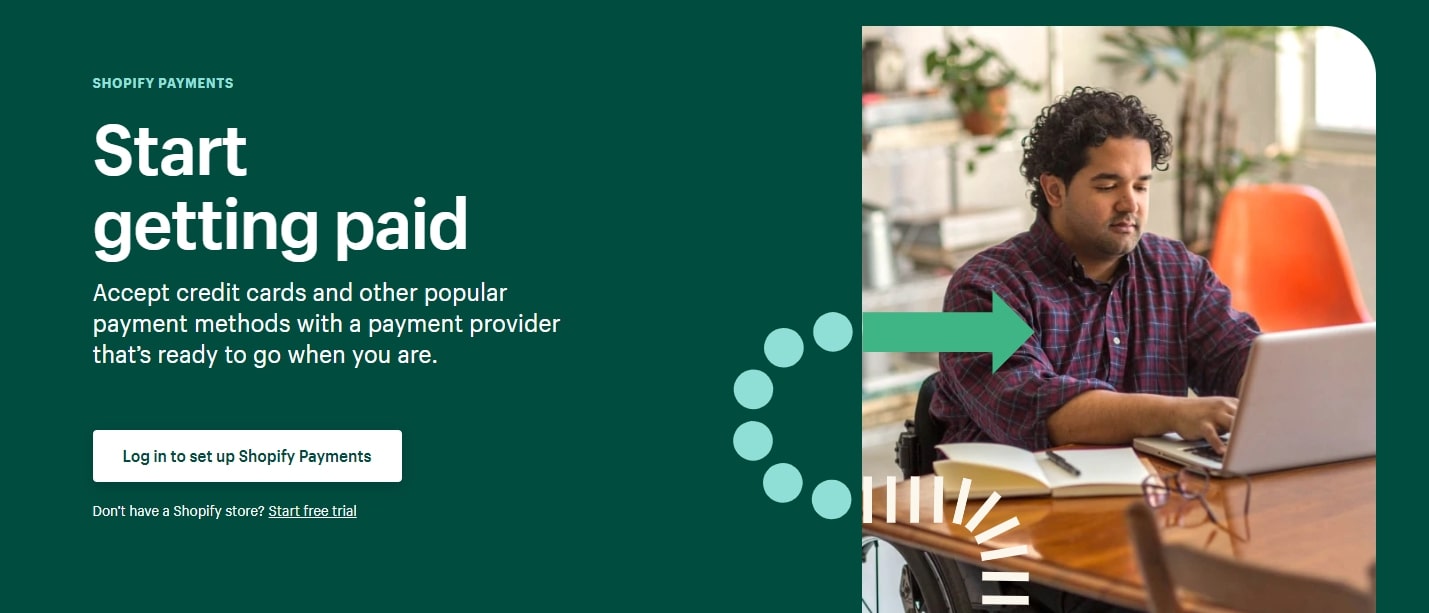**Caption:**

This detailed Shopify advertisement showcases a professional landing page designed to entice potential users to set up Shopify Payments. The background is a dark green hue, creating a striking contrast to the central elements.

On the right side of the layout, there's a photograph featuring a man in his early 30s with curly hair and a plaid shirt. He is seated at a desk, engaged with an open book and using a laptop. The setting appears cozy and professional, adorned with plants, a window, chairs, and additional office decor in the background.

Adding a subtle yet engaging visual touch, there are dashed lines originating from the lower left-hand corner of the image. These lines transition into circles that outline the photo and curve back, transforming into a teal arrow that overlays the image.

In the upper left-hand corner, a green field contains marketing text in various fonts and sizes. The text begins with "Shopify payments" in small, lightweight lettering, followed by the larger, bolder phrase "Start getting paid." The subsequent smaller text encourages users to accept credit cards and other popular payment methods with a readily available payment provider. The call-to-action button states "Log in to set up Shopify payments," and an additional link beneath it offers a free trial for those without a Shopify account, rendered in white, underlined text.

The text is left-justified, with "start" inexplicably placed on its own line, differing from the rest of the message. Notably, the upper right-hand corner of the man's photo has a rounded edge, while the remaining corners are squared off.

This image captures a polished and professional look, though it is unclear if additional content may be present beyond the screenshot provided.